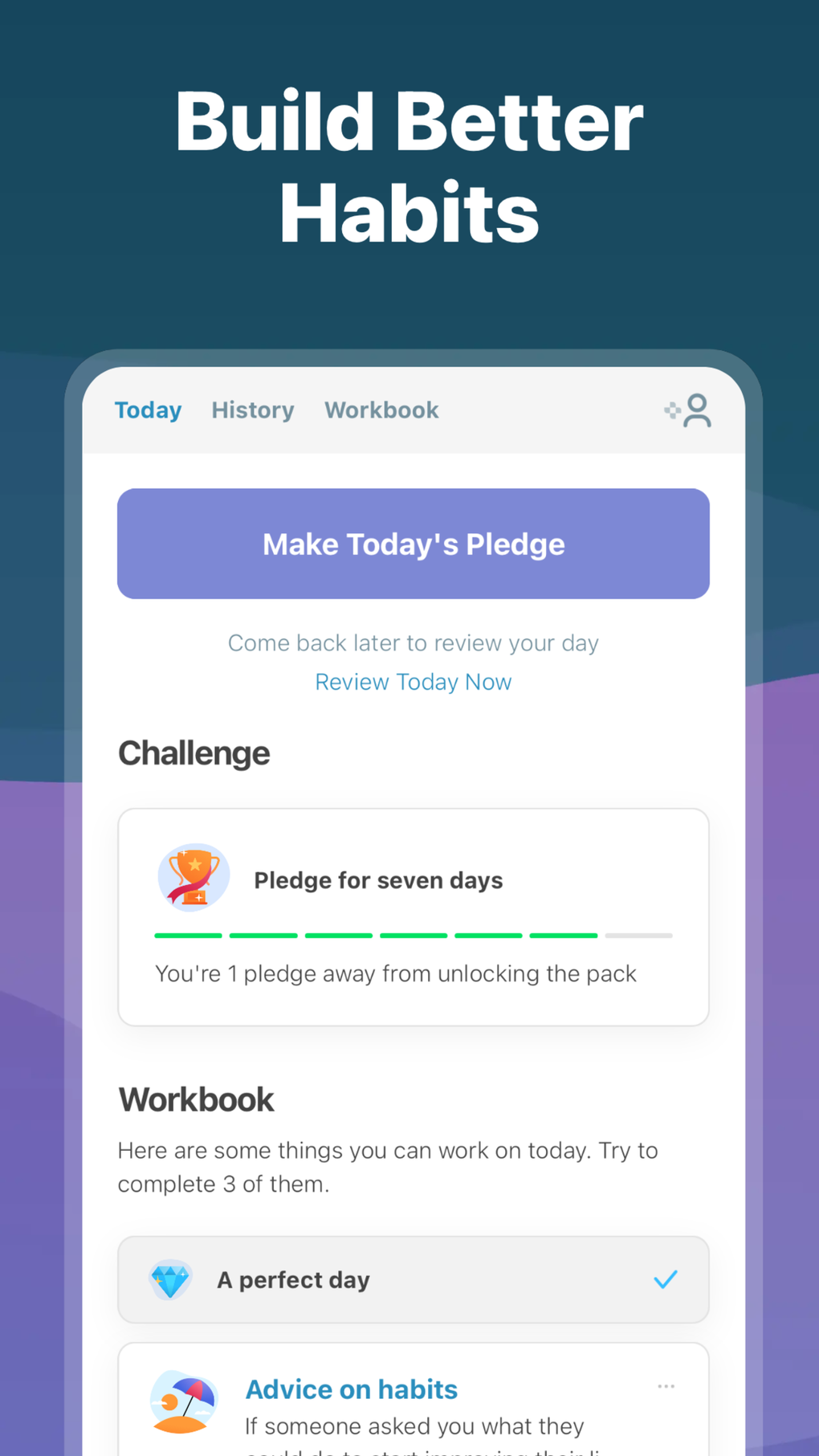This image is a promotional screenshot for a habit-building application. At the top, in large centered white letters, the headline reads "Build Better Habits." Below the headline, a simulated phone screen is displayed, showing various sections of the app interface. 

At the top of the phone screen, there are three tabs labeled "Today," "History," and "Workbook," with "Today" being highlighted. Centered just below these tabs, a prominent button encourages users to "Make Today's Pledge." Underneath this button, a message prompts users to "come back later to review your day" with a hyperlinked option to "Review Today Now."

Further down, the interface features a section labeled "Challenge" on the left, advising users they are just one pledge away from unlocking a reward pack for pledging for seven consecutive days. Next, a "Workbook" section offers tasks to complete, urging users to try to finish three activities for the day.

A banner, adorned with a diamond icon and a check mark, highlights an achievement titled "A Perfect Day." Finally, there is a snippet of a section labeled "Advice on Habits," though the rest of the screenshot is partially cropped.

The lower portion of the screenshot has a purple background, suggesting it could be part of a series of images or an advertisement for the app.